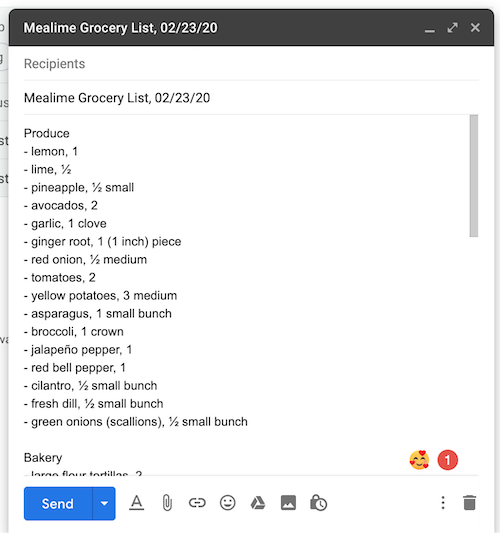This image is a screenshot of a grocery list taken on February 23rd, 2020. The screenshot itself contains a gray stripe running diagonally from the upper left to the lower left, partially obscuring the words "G" and "S" and "ST." The purpose of the screenshot is to display the grocery list titled "Mealtime Grocery List."

Underneath the title, "Mealtime Grocery List," the list is divided into sections:

**Produce:**
- One lemon
- Half a lime
- Half a small pineapple
- Two avocados
- One clove of garlic
- One-inch piece of ginger root
- Half medium red onion
- Two tomatoes
- Three medium yellow potatoes
- One small bunch of asparagus
- One crown of broccoli
- One jalapeno pepper
- One red bell pepper
- Half a small bunch of cilantro
- Half a small bunch of fresh dill
- Half a small bunch of green onions (scallions)

The next section is titled "From the Bakery." The text is slightly cut off by the need to scroll down, revealing partially "Large flour tortillas too..."

On the upper right-hand side of the screenshot, there is a gray vertical scrollbar indicating that more information is available by scrolling down. In the bottom right corner, there is a happy emoji expressing affection, suggesting the person who took the screenshot is pleased or grateful for the list. The bottom left corner contains a button to send the list, allowing it to be shared with others.